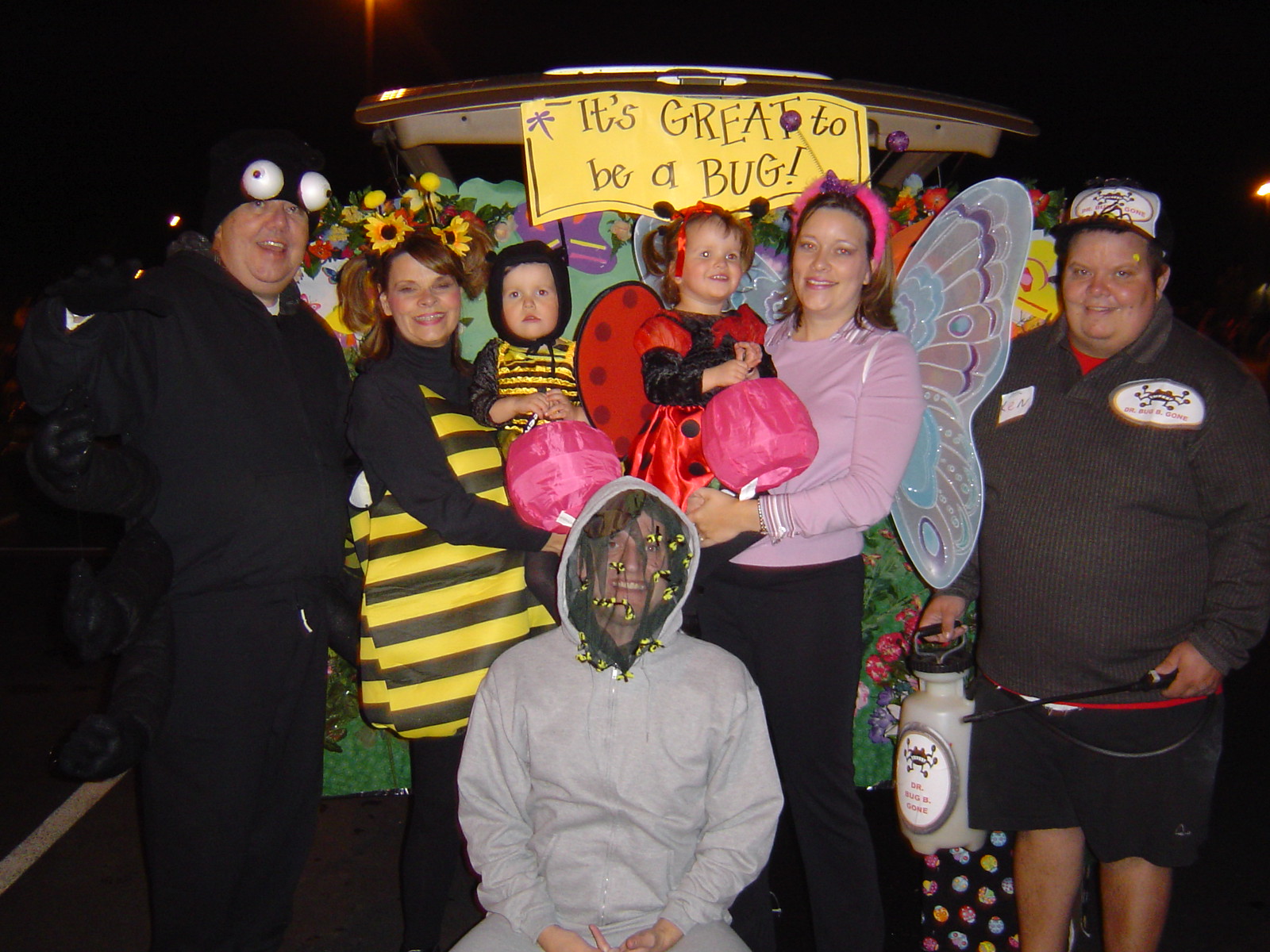In the image, a group of seven people pose in a parking lot at night, all gathered under a yellow sign that reads "It's Great to Be a Bug" in handwritten black text, surrounded by a thin black border. The central focus is on two women holding children, each dressed in coordinated costumes. One woman and her child are both adorned in bumblebee outfits, with the woman sporting sunflowers on her headgear. Beside them, another woman, dressed as a butterfly with wings reminiscent of an angel, holds a girl in a ladybug costume. Both children carry pink baskets, suggesting a Halloween setting. Flanking the women are men in dark clothing; the man to the right wears a dark jacket and pants with a hat featuring big white bug eyes, while the man to the far left is dressed more casually in a red t-shirt under a gray sweater, black shorts, and a hat. A child in the front, dressed in a white hoodie with a net over their head adorned with yellow specks, smiles and kneels, embodying another bug-themed attire. The group’s joyful camaraderie and costumes hint at a bug-themed festival or Halloween celebration.